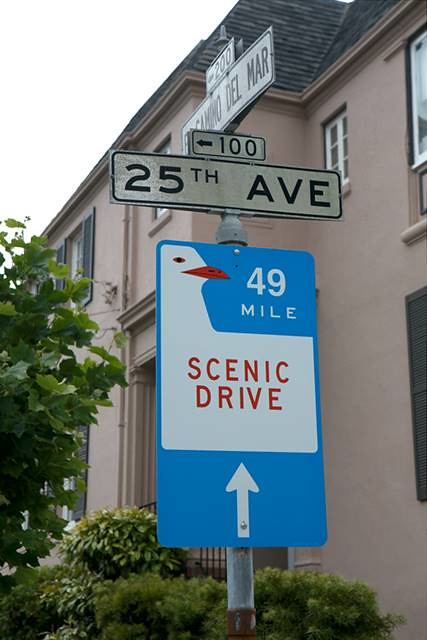In this image, the central focus is a collection of street signs mounted on a single pole, standing against an urban backdrop. The background features a grayish pink building with several windows and a black slate roof, providing a subtle contrast to the foreground elements. In front of the building, lush bushes and potentially a tree with visible leaves add a touch of greenery to the scene.

The street signs, positioned prominently in the center, include a sequence of rectangular signs. At the bottom, a large, bright blue sign with a seagull design reads "Scenic Drive" in red lettering. An upward-pointing arrow and the text "49 Mile" in white occupy the top right corner of this sign. Directly above, a white rectangular sign states "25th Avenue." Higher still, a smaller sign features an arrow pointing left alongside the number "100." At the very top, perpendicular to the "25th Avenue" sign, another street sign, slightly harder to read, likely says "El Camino del Mar," accompanied by an arrow pointing left and the number "200" in a smaller rectangle just above it.